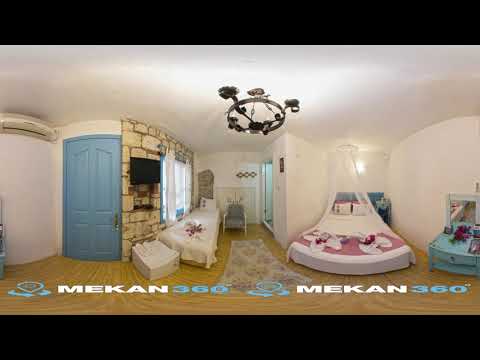The image depicts a distorted panoramic view of a bedroom, accentuated by a wide-angle lens that rounds and stretches the perspective. The scene features white walls and a variety of furniture. To the right, there's a distinctive bed with a white bedspread, a pink blanket at the base adorned with white decorations, and a white lace canopy, giving it a somewhat triangular shape due to the lens distortion. A teal vanity is situated in the lower right corner. 

On the left side of the room, a blue door stands out next to a stone light brown wall, which hosts a mounted TV. In this area, there is a daybed with a white bedspread and a small gray chair nearby. The flooring appears to be either wooden or tiled, though the pattern is unclear due to the distortion.

The photograph has black bands on the top and bottom, overlaid with branding text. The text reads "MEKAN 360" in white and turquoise letters, accompanied by a robin’s egg blue logo. A black chandelier hangs from the white ceiling, adding to the room's atmosphere. The overall impression is that of a showroom or a catalog display for Mekan 360 furniture.